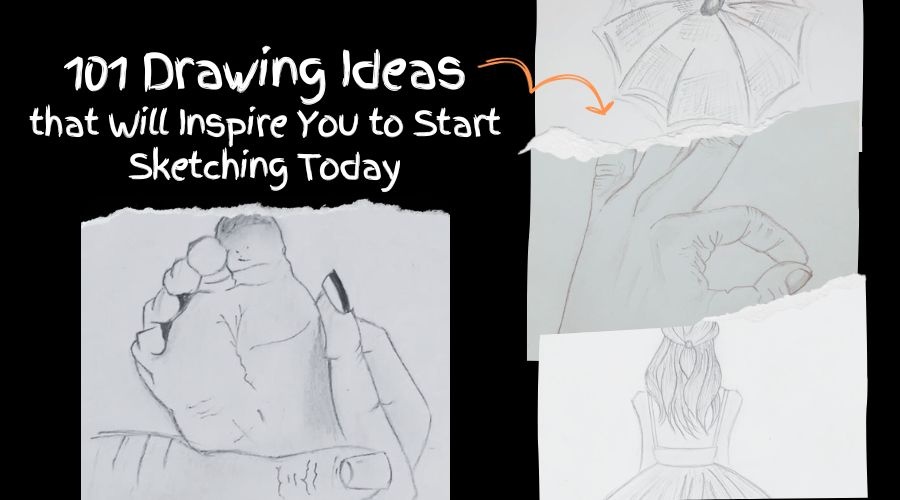The image is a horizontally rectangular, black-and-white photograph with no border. The background is pure black, creating a striking contrast with the light gray paper drawings. In the upper left corner, hand-drawn white text reads, "101 Drawing Ideas That Will Inspire You to Start Sketching Today." An orange arrow links the word "Ideas" to a sketch of an umbrella on another piece of paper. The image features four pencil drawings on torn paper. On the top right, there is an umbrella drawn from above. Below it, there is a sketch of a left hand making the OK symbol. At the bottom right, there is a rear view of a girl with her hair put up, wearing a long dress. On the left side, there is a drawing of a baby's foot being gently held by an adult hand, showcasing detailed depictions of the hands and the foot, complete with visible toes.